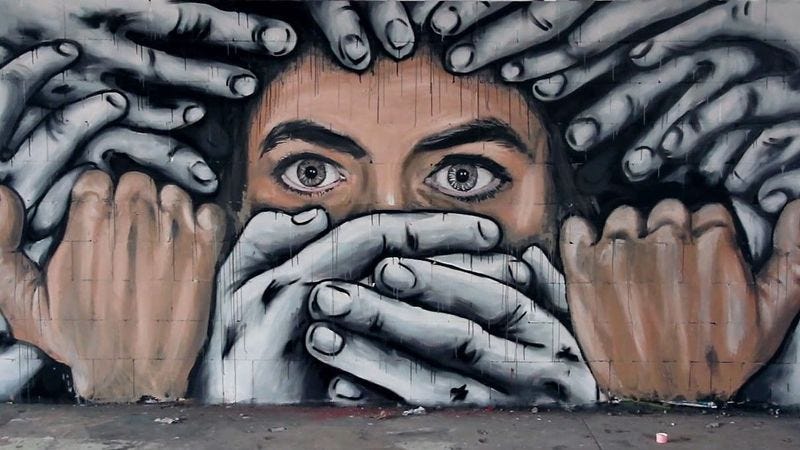This image showcases a dramatic and dynamic mural painted on the side of a building. The artwork, predominantly in black and white with hints of skin tone, centers on a large, expressive face of a person, possibly a woman. Her wide, intense eyes and black eyebrows peer out from the mural, framed by her black hair and contrasting white skin. Gray, almost ghostly, fingers and hands surround and interact with her head, creating a sense of tension and movement. Some of these gray hands seem to be grabbing or consuming her, with two specifically covering her mouth, intensifying the dramatic effect. Her own hands, which are light brown and colored distinctly from the gray, are positioned on either side of her head as though trying to fend off the invasive, gray hands. This powerful scene is set against the backdrop of a concrete sidewalk littered with trash, adding to the gritty and somber atmosphere of the mural.